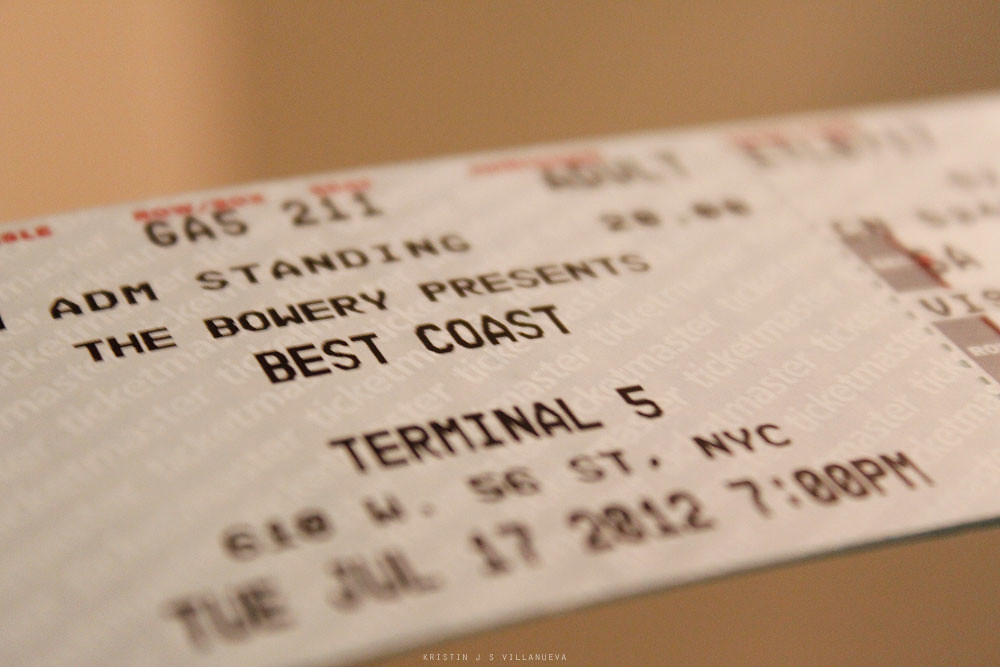This image features a close-up photograph of a concert ticket for Best Coast at Terminal 5 in New York City. The ticket, positioned on a reflective brown surface, shows clear details in the middle while the edges are blurred. At the very top, it reads "GA5-211" and "ADM standing $26.00." Below this, it states "The Bowery Presents Best Coast" and "Terminal 5," with the venue's address "610 W. 56th Street, NYC." The ticket is for the event on Tuesday, July 17, 2012, at 7 p.m. The pinkish ticket has perforations for the stub, and the background reveals a repetitive "Ticketmaster" logo, suggesting it is printed on an official Ticketmaster paper.